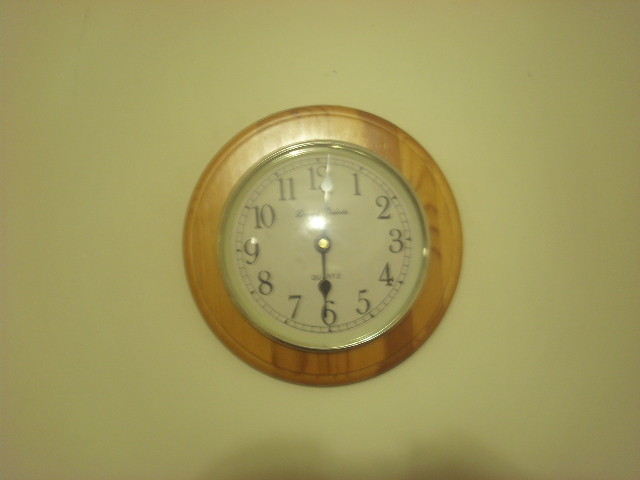This photograph captures an analog clock mounted on a cream-colored painted wall. The clock features a classic design with a white face and black numerals ranging from 1 to 12. The hour and minute hands are also black, indicating the time as two minutes past six. Surrounding the clock face is a golden-colored border, which is encased in a 1 to 2 inch thick wooden frame. The flash from the camera has caused a glare on the glass covering the clock, making it difficult to discern the fine details, including some lettering that likely represents the clockmaker's name.